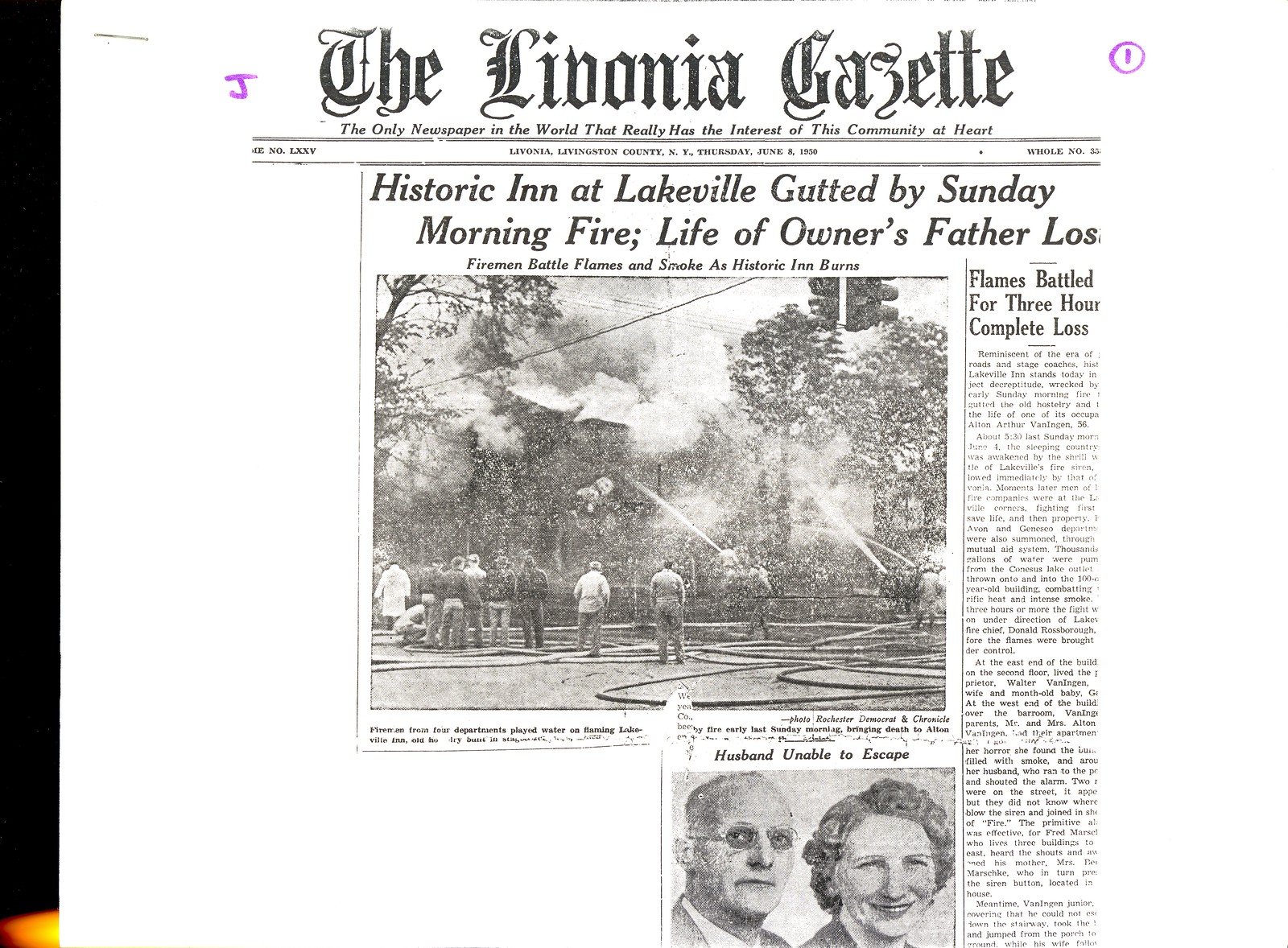The image is a wide rectangular scan of a newspaper, featuring several distinct elements. On the left side, there is a vertical black rectangle with an orange bottom. The rest of the image showcases a piece of an old newspaper with an off-white background. In the top left corner, a purple marker denotes a "J," while the top right corner has a circled "1." The newspaper's title, "The Livonia Gazette," is prominently displayed at the top, followed by the tagline: "The only newspaper in the world that really has the interest of this community at heart."

An eye-catching photograph takes center stage, depicting several men wielding hoses and battling a significant blaze consuming a house. Surrounding trees also appear to be on fire. The headline accompanying this dramatic image reads: "Historic Inn at Lakeville Gutted by Sunday Morning Fire. Life of Owner's Father Lost." The chaotic scene indicates that flames were battled for three hours, leading to a complete loss.

Below the main article and photograph, there is another image of a middle-aged couple, presumably in their 50s or 60s, with the caption "Husband Unable to Escape." The lead story details the unfortunate event, mentioning that the life of the owner's father was claimed in the inferno. The text of the article itself is partially obscured, hinting that part of it may have been cut off or is too small to decipher. Overall, the newspaper page illustrates a tragic event that deeply affected the community, capturing both the intense firefighting efforts and the personal loss suffered by the family.